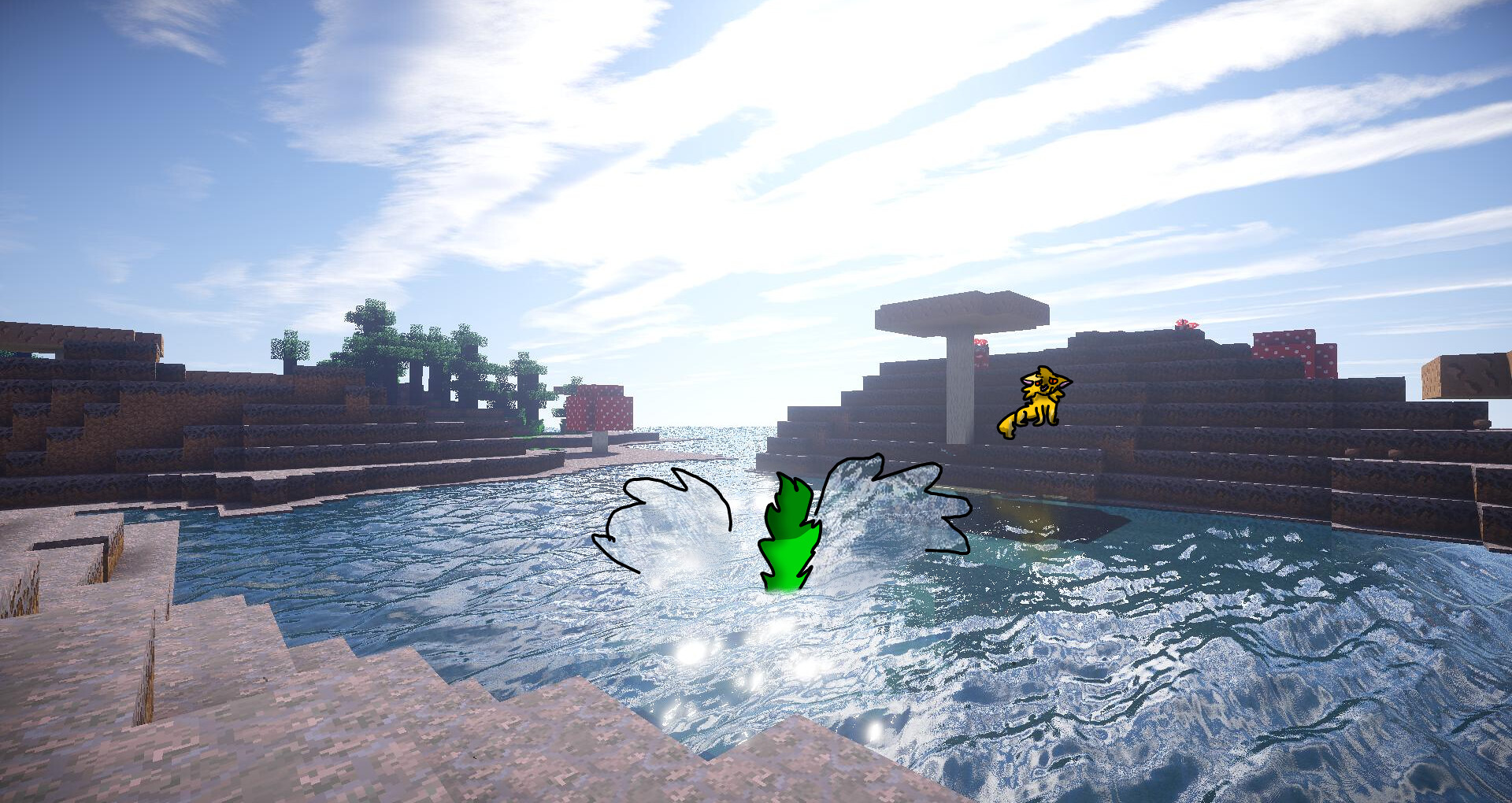A digitally-crafted image showcases an opulent, unusually designed pool area. The scene features a large, elaborate swimming pool surrounded by an array of oddly-shaped, rectangular structures. These structures, positioned on all sides of the pool, vary in color and form, diverging significantly from conventional poolside architecture. In the foreground, primarily to the left and bottom, there are blocks in shades of pink and gray. Rows of darker brown blocks are seen in the middle sections to both the right and left of the pool.

Above the bleachers, an enigmatic pedestal or stand is present, possibly meant to hold people or objects, though its exact purpose remains unclear. Adding to the surreal nature of the image, a cartoon-like element is included: a bright green flame, depicted with black ink squiggles and emitting a splash pattern, appears to enter the water. Emerging from this green flame is a whimsical lion character, further contributing to the image’s fantastical and ambiguous narrative.